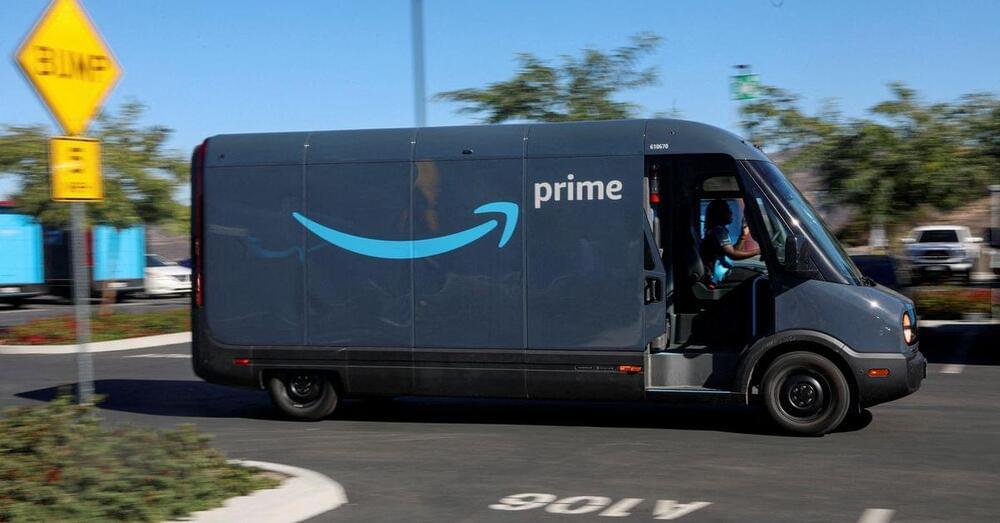A vibrant, high-resolution digital screenshot captures a dynamic outdoor scene under a stunning baby blue sky. In the slightly blurry background, indicative of motion, lush green trees line the landscape, with one prominent tree on the left, one near the center, and two more on the right side. A white pickup truck is visible in the background on the right, while on the left side, a diamond-shaped sign with "BUMP" in bold black letters stands out against its white and yellow background. Below it, a yellow square sign subtly reads "5 MPH," though the "MPH" is barely legible. Evergreen bushes occupy the bottom-left corner, bordered by a gray concrete curb and black asphalt. Just to the left of center, an upside-down parking spot marker displays "A106" in white.

The focal point of the image is an Amazon Prime van, painted in a dark blue hue. The vehicle is moving to the right, its open door revealing a Black gentleman either entering or exiting the van, with his arm clearly visible. The Amazon logo, a light blue arrow that curves downward before pointing up, adorns the side of the van. The word "Prime" is emblazoned in white on the right side, near the open door, accentuating the brand identity. This dynamic shot beautifully combines elements of nature and urban life, capturing a moment of everyday activity with remarkable clarity.